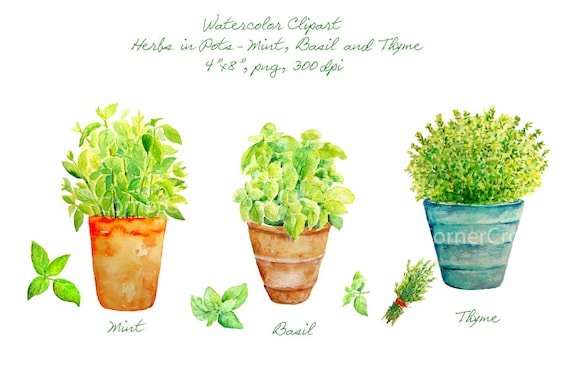This watercolor illustration beautifully depicts three pots of herbs arranged from left to right: mint, basil, and thyme. Each plant is meticulously detailed, with both the pot and the plant itself rendered in rich, vibrant colors. The mint is planted in a terracotta-colored pot with the label "mint" underneath it, accompanied by a close-up of a mint leaf to its left. The basil, placed in a similarly terracotta-colored pot, is labeled "basil" in cursive beneath it and features additional basil leaves both to the left and right of the pot. The thyme, distinguishable by its blue pot with horizontal stripes, has "thyme" written underneath and includes a sprig of thyme tied with a red ribbon on the left. At the top center of the image, the text "Watercolor Clip Art. Herbs in Pots - Mint, Basil, and Thyme. 4x8 PNG 300 DPI" is prominently displayed, adding to the professional presentation of this detailed artwork.